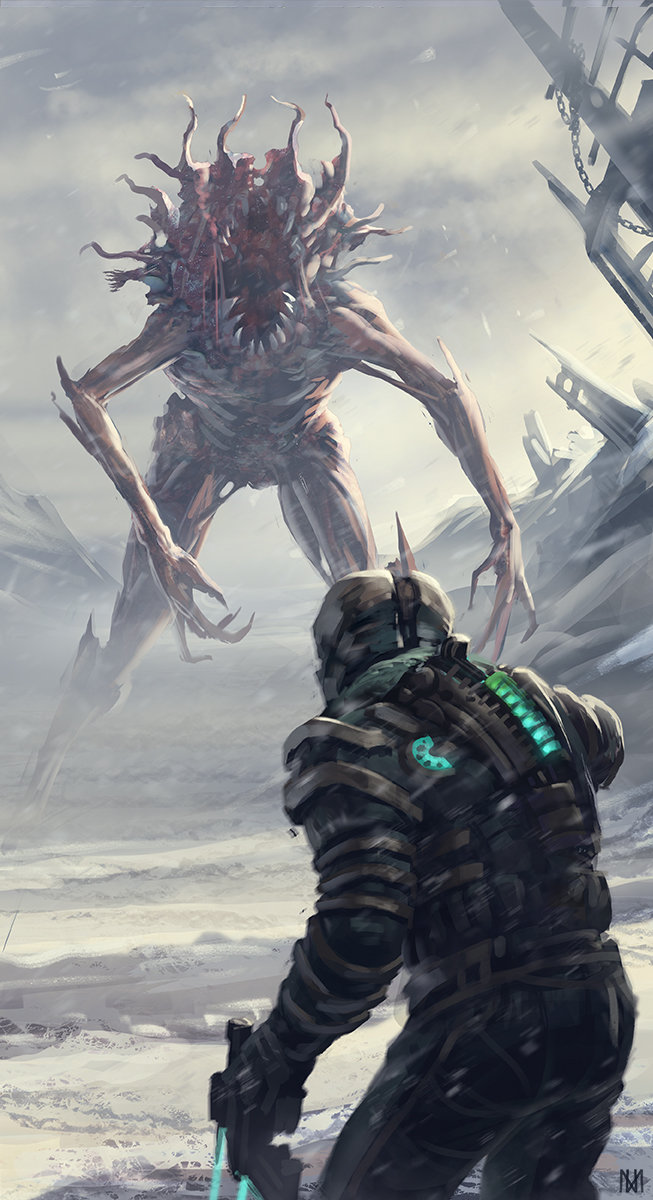This detailed and artistic poster, reminiscent of a science fiction or fantasy setting, shows a dramatic scene on a snowy surface. Dominating the top center is a monstrous creature, facing the viewer with an imposing presence. In contrast, at the bottom right corner, a smaller character, clad in green with some sort of metal protection, stands with their back to us. Their fingers are extended into saber-like shapes, hinting at a supernatural or superhero nature. The scene is enveloped in a palette of white, gray, black, light blue, brown, tan, red, and turquoise, with an indistinct, snow-covered background that contributes to the image's mysterious and otherworldly ambiance. No text accompanies the image, heightening its enigmatic appeal, making it feel like a poster for a video game, movie, or comic book.